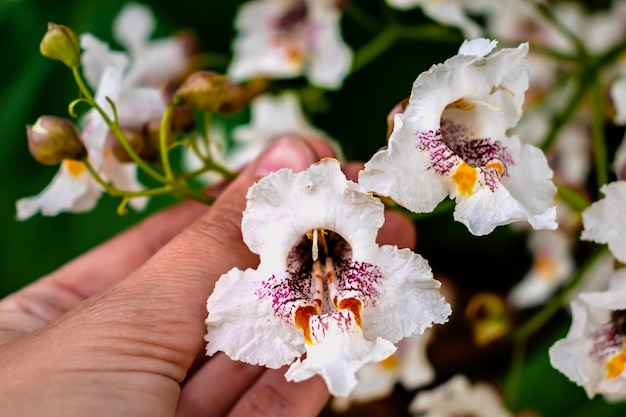The image depicts a close-up of a hand, belonging to an unidentified individual, delicately holding the stem of a small cluster of white flowers that are still attached to the bush. The focal point is a prominent white flower with three larger petals. The flower's center features deep purple tendrils radiating outward, complemented by dark yellow, almost golden splotches. Alongside the main flower, still attached to the same green stem, are several unopened buds on the left and about 8 or 9 more similar flowers in various stages of bloom. The background features a gradual blur, showcasing more of these elegant white flowers with their distinctive purple and yellow centers, enhancing the depth and focus on the primary flower held between the person's fingers.